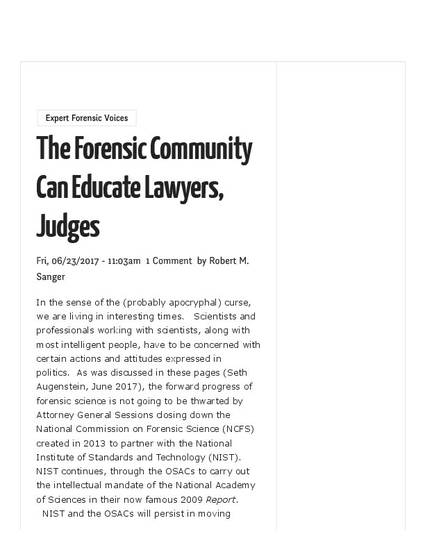**Caption:**

This image features an article, presumably from a newspaper, entitled "Expert Forensic Voices," prominently displayed in a rectangular heading at the top. The text is set against a white background with black print. The article's headline reads, "The forensic community can educate lawyers, judges," followed by the date "Friday 06/23/2017 - 11:03 AM" and a note indicating one comment by Robert M. Sanger.

The article opens with a philosophical reflection, "In the sense of the probably apocryphal curse, we are living in interesting times," before delving into the implications of recent political actions on forensic science. It highlights the concerns of scientists and professionals in the face of politicized decisions, specifically referencing Attorney General Sessions' closure of the National Commission on Forensic Sciences. Created in 2013 to coordinate with the National Institute of Standards and Technology (NIST), the commission's dissolution poses challenges. However, the article reassures that the forward progress of forensic science will not be thwarted. NIST, through its Organizational Scientific Area Committees (OSACs), remains committed to the intellectual mandate set forth by the National Academy of Sciences in their pivotal 2009 report. The article concludes abruptly, with a final note on NIST and the OSACs' continued efforts being cut off.